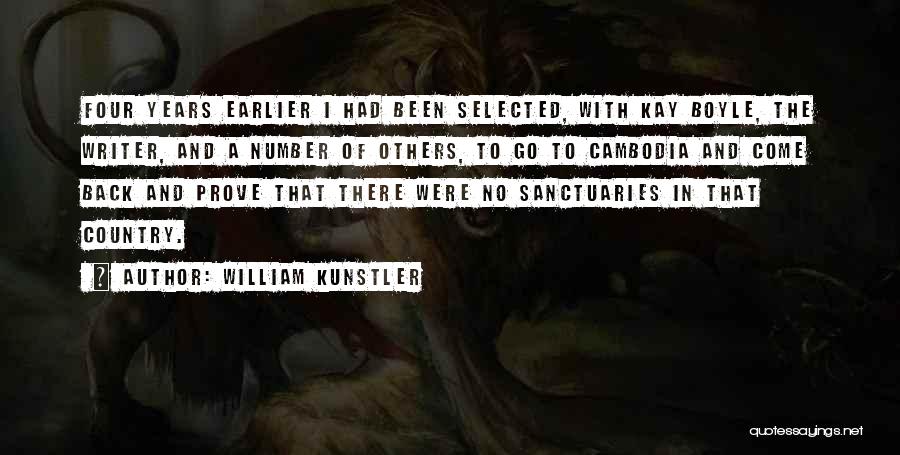The image depicts a dark, almost shadowy animal, possibly a bull or lion, set against a predominantly black background. The central area of the image features a series of slightly grungy white rectangular strips, arranged in a column, each containing black stamped text. The text reads: "Four years earlier I had been selected with K. Boyle, the writer and a number of others to go to Cambodia and come back and prove that there were no sanctuaries in that country?" This quote is attributed to author William Kunstler, with the attribution included on the final strip. The bottom right-hand corner bears the website name "quotesayings.net". The dark and ambiguous nature of the background, combined with the layered text, gives the image a mysterious and slightly unsettling appearance.